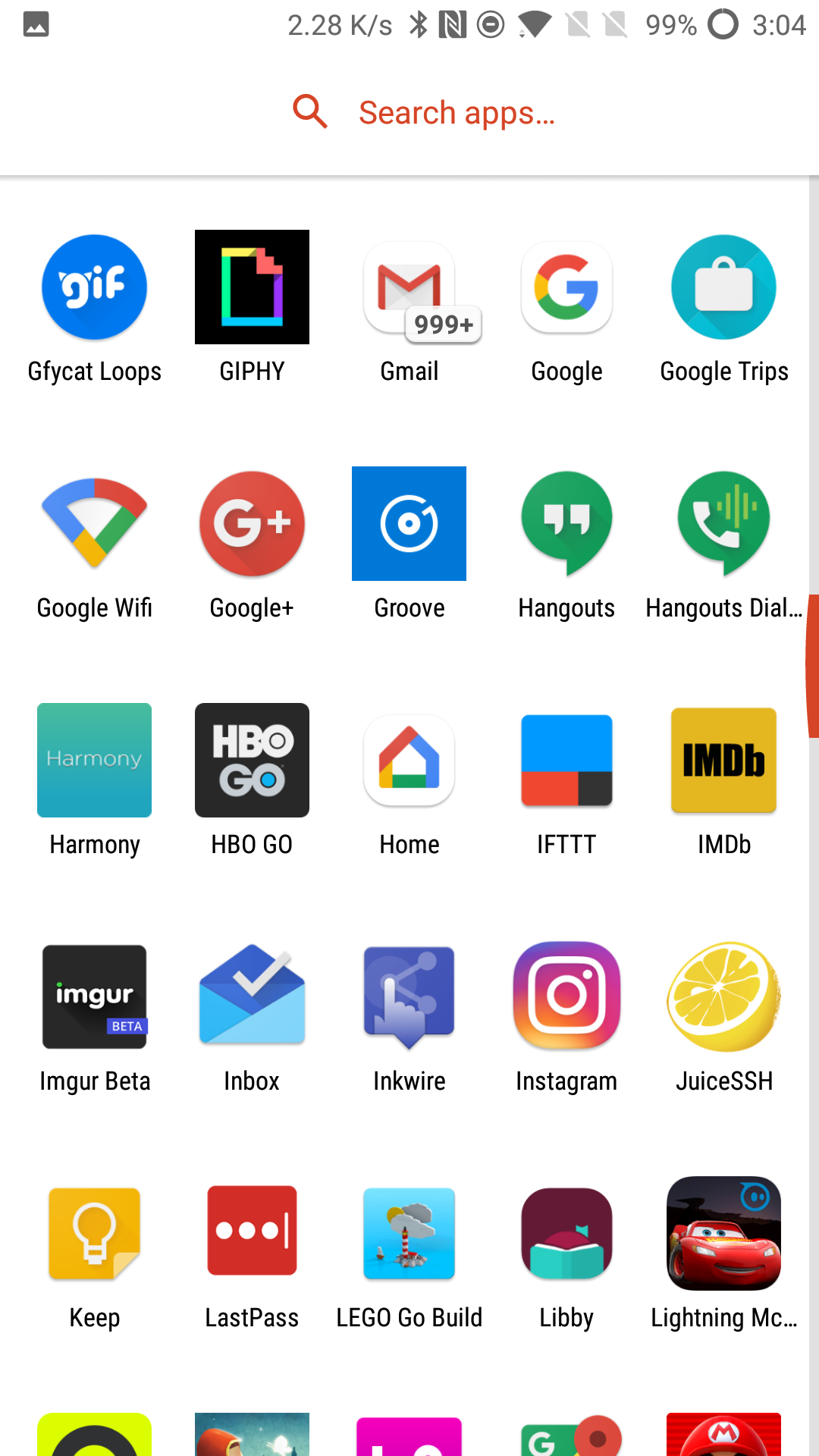This detailed screenshot from a smartphone displays its app menu. At the top right corner, the status indicators show "2.28k/s", indicating a data rate, along with icons for Bluetooth, Wi-Fi, and battery life at 99%. Below this, the search bar labeled "Search apps" is present. The list of visible apps includes:

- GFYCat Loops
- Giphy
- Gmail (with a notification icon showing "999+" unread emails)
- Google
- Google Trips
- Google Wi-Fi
- Google Plus
- Groove
- Hangouts
- Hangout Style
- Harmony
- HBO Go
- Home
- IFTTT
- IMDb
- Imgur Beta
- Inbox
- Inquire
- Instagram
- JuiceSSH
- Keep
- LastPass
- LEGO Go Build
- Libby
- Lightning McQueen

The screenshot is wider than it is tall, cutting off some apps at the bottom edge, making them illegible. There are no people, animals, or plants in this image.